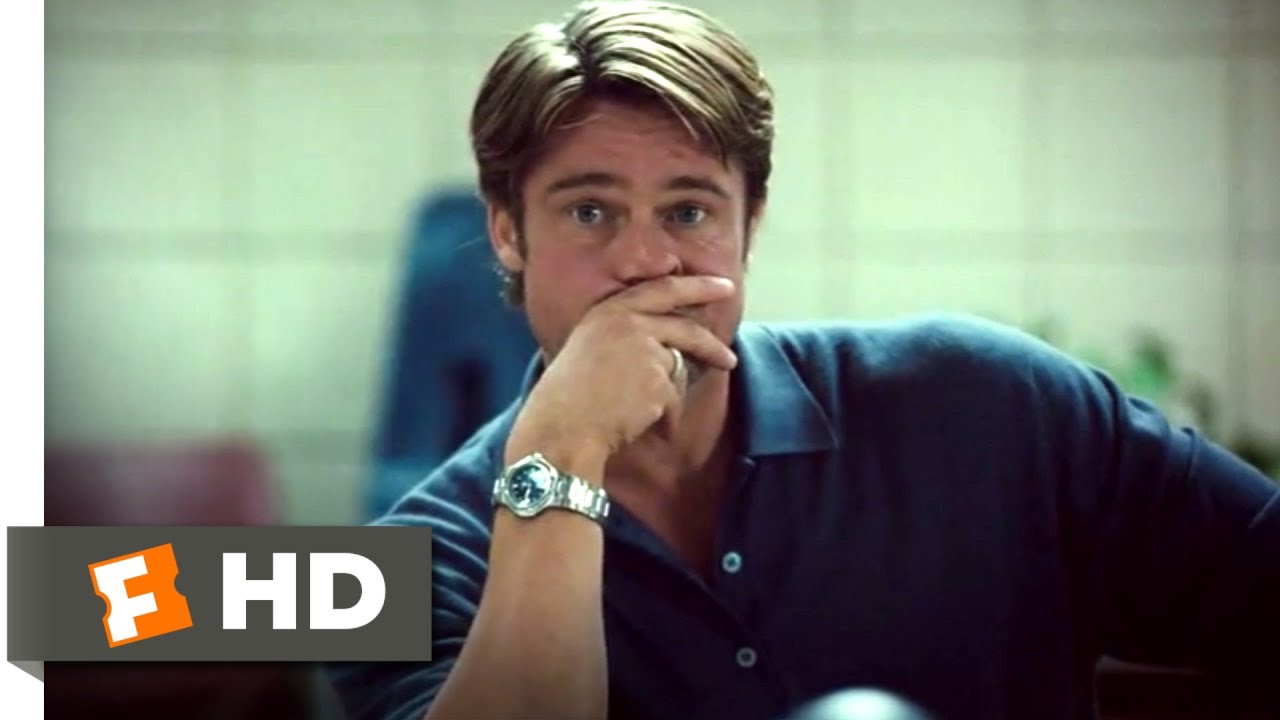In this detailed photograph, a young Brad Pitt is captured looking directly into the camera with a somewhat shocked expression. His light brown hair is parted and falls just short of his ears. He is clad in a blue polo shirt with a button placket. His left hand, adorned with a gold wedding band, covers his mouth just beneath his nose, while his right hand, featuring a silver watch with a blue face, rests on the table or desk in front of him. The background is a white wall with a beige tone that appears out of focus, and a blue object can be seen behind him. The image features a prominent logo in the bottom left corner, consisting of an orange square with a white "F" and large white "HD" lettering next to it. The position of Brad Pitt is central within the frame, adding to the intimate, direct nature of the shot.